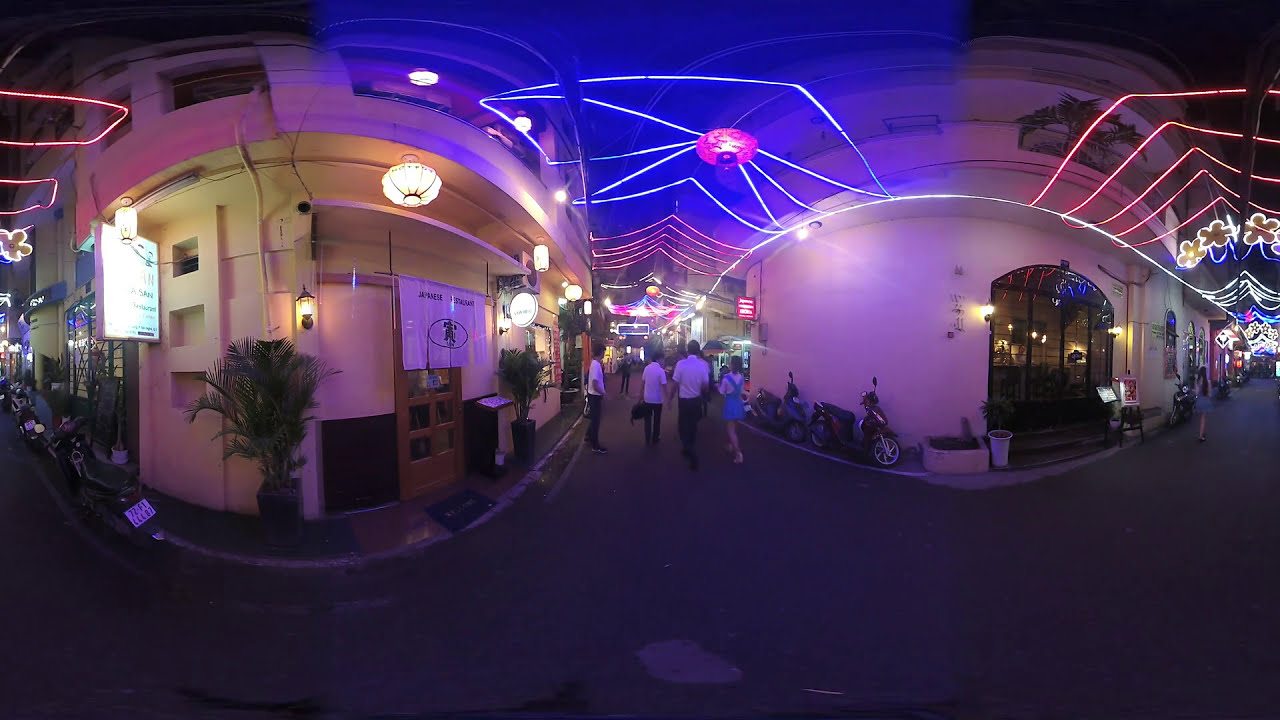This captivating nighttime photograph captures a bustling urban scene, possibly an Asian street market, showcasing a vibrant alleyway or sidewalk situated between two light-colored buildings. The image, likely taken with a fisheye lens to create a unique curvature effect, reveals a dark gray walkway adorned with neon glowing lights and decorative lanterns strung overhead, forming an inviting archway that illuminates the corridor. In the foreground, a group of people dressed in white shirts and dark pants strolls down the center pathway, accompanied by a woman in a blue dress with a cross-shaped back, partially covered by a white shirt underneath. To the right, a row of parked scooters fronts a building that appears to be a restaurant, as suggested by the visible doorway and foreign language symbols around the stores. The scene, rich with cultural decor and vibrant light, encapsulates the lively and enchanting atmosphere of a night market in a foreign land.